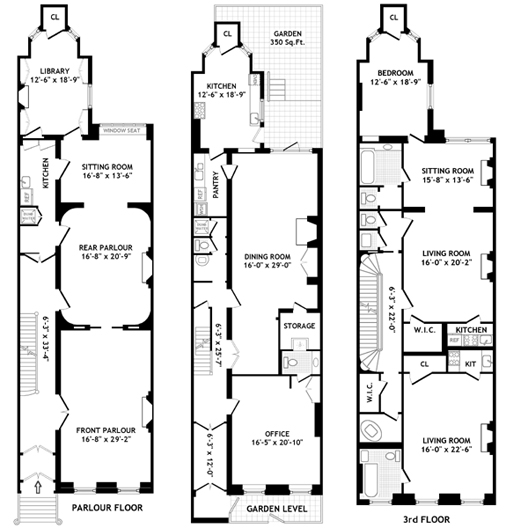This image showcases a detailed floor plan of a three-story house, meticulously lined and labeled in black ink. The first floor, referred to as the parlor level, includes rooms such as a library, kitchen, sitting room, rear parlor, and front parlor, each accompanied by specific dimensions. Moving to the second floor, known as the garden level, the layout features a kitchen, pantry, dining room, office, and storage, also marked with precise measurements. This level also includes access to a garden. The third floor depicts a layout consisting of a bedroom, sitting room, living room, secondary living room, and another kitchen, all with their respective dimensions clearly indicated. Each room and structural element, including walls, doors, windows, and stairs, is intricately detailed, providing a comprehensive view of the house's layout.